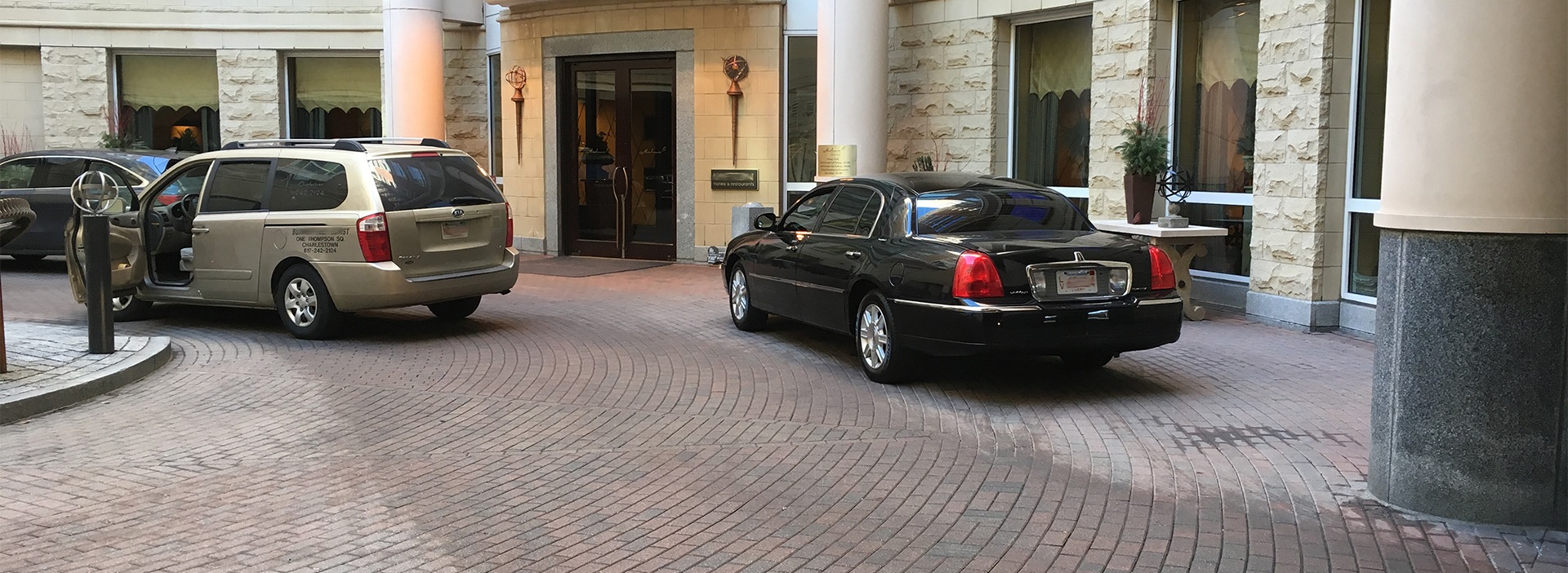This image depicts the exterior of what appears to be a grand hotel or restaurant, featuring a circular driveway paved with bricks. The impressive building, constructed from stone painted in a whitish-yellow or eggshell hue, showcases large cylindrical columns that flank the towering front door, which is likely over 10 feet tall. Decorative elements include metal swords attached to globes on either side of the entrance. To the far right, a massive green marble base supports an equally grand column extending out of the frame.

Three vehicles are prominently parked within the circular drive. A sleek black town car, noticeable by its red taillights, is parked to the right. Positioned to the left is a beige minivan with its driver's side door ajar. Slightly further to the left, a partially visible SUV or van is situated near the top left corner of the image. The windows of both the building and the cars appear to be tinted, obscuring any view inside.

The scene captures the atmosphere of late evening or an overcast day, with ambient lighting creating a faint orange glow from the building. A small, green sign near the door hints at the establishment's identity, though its text is unreadable from the camera's perspective. Stretching about 50 feet away, the camera angle reveals a potentially wet or dirty band down the middle of the brick driveway, while the surrounding areas remain dry.

In the background, large windows interspersed with structural concrete elements extend across the façade, contributing to the stately appearance. A person may be standing near the minivan, though this detail is unclear. Additional writing on the beige van reads "1 Thompson Square, Charleston," with an associated phone number, reinforcing the upscale ambiance of the setting.